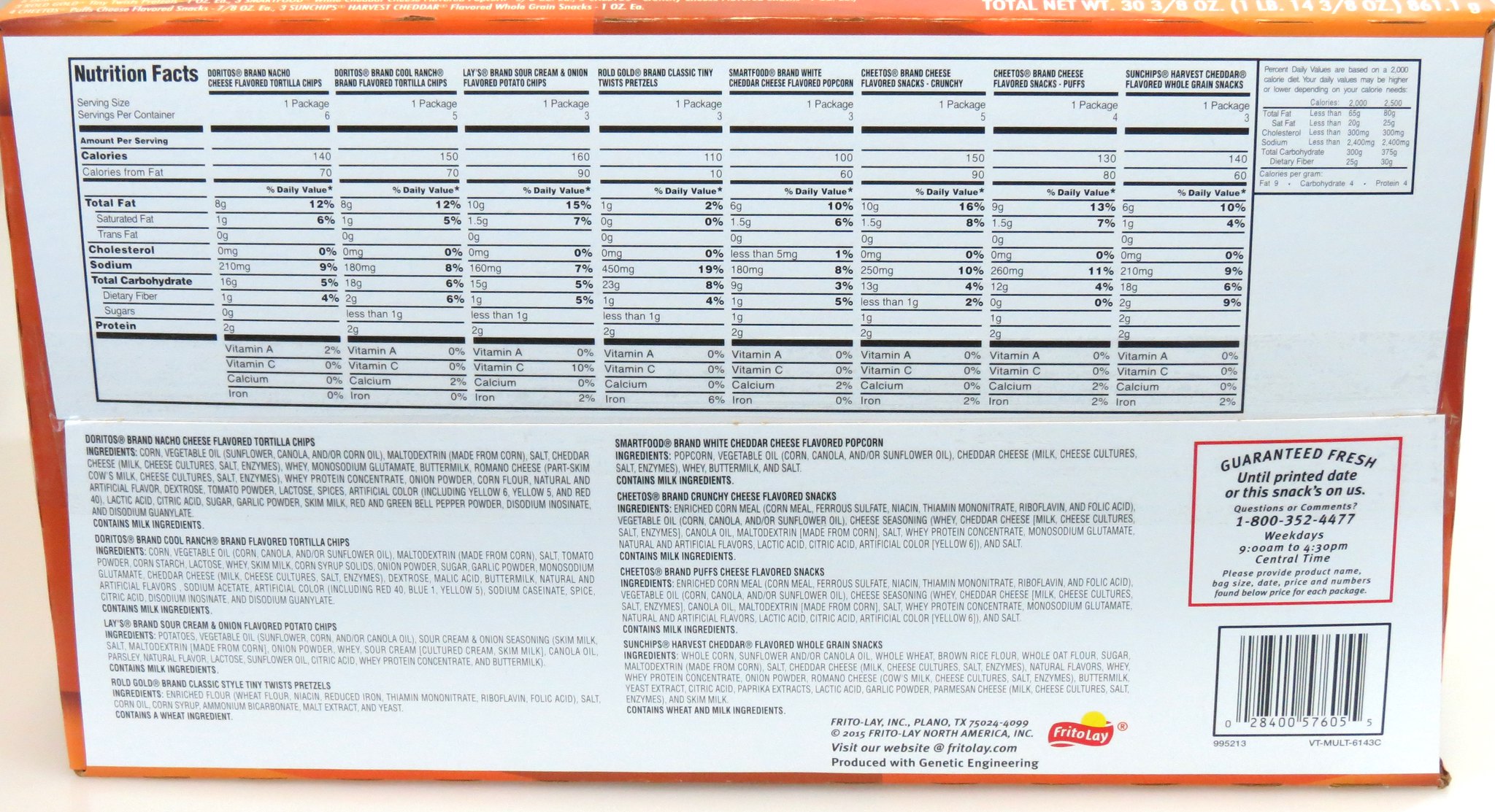This photograph features a multi-pack of Frito-Lay products, prominently showcasing a large and detailed Nutrition Facts label rendered in white with black font. The main packaging, displayed in various shades of orange, highlights several flavors within the pack, though specific details are obscured due to the graininess of the image. A comprehensive ingredients list is also visible on the back of the package. White font adorns the front of the package, which also features a barcode, a "Guaranteed Fresh" square, and a customer service phone number, albeit too distant to be read clearly.